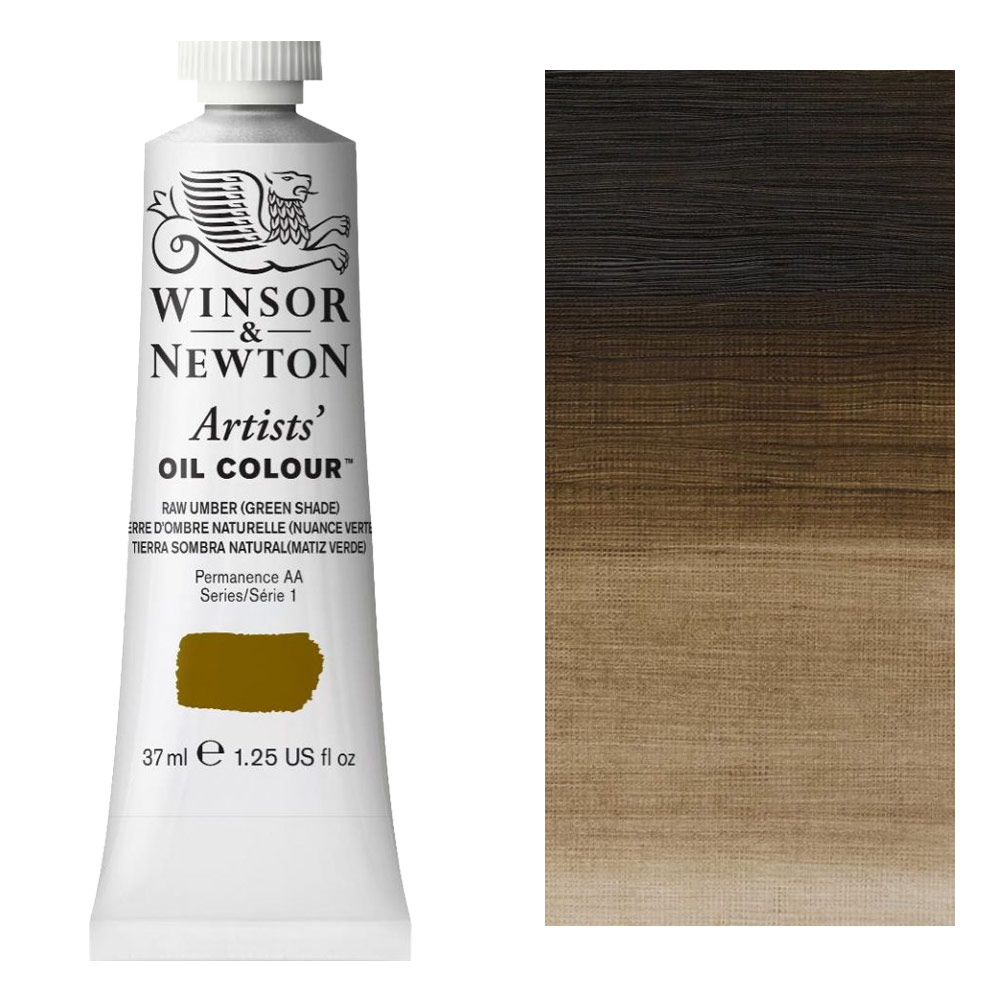The image features a detailed product photo of Winsor & Newton Artist's Oil Color in the shade of Raw Umber (Green Shade), showcasing an aluminum tube with a white, ridged screw cap. The text on the tube includes the brand name, product line, and color designation, with translations in French and Spanish. The permanence is rated AA, and it is part of Series 1. The tube displays a brushstroke-shaped swipe of the color, which is solid and dark brown. The volume is labeled as 37 milliliters (1.25 US fluid ounces). Positioned on the left side against a white background, the tube is complemented on the right by a tall rectangular sample displaying the paint’s varying thicknesses on either canvas or wood texture. The sample transitions from a rich dark brown to a lighter tan, illustrating the range of the raw umber shade.